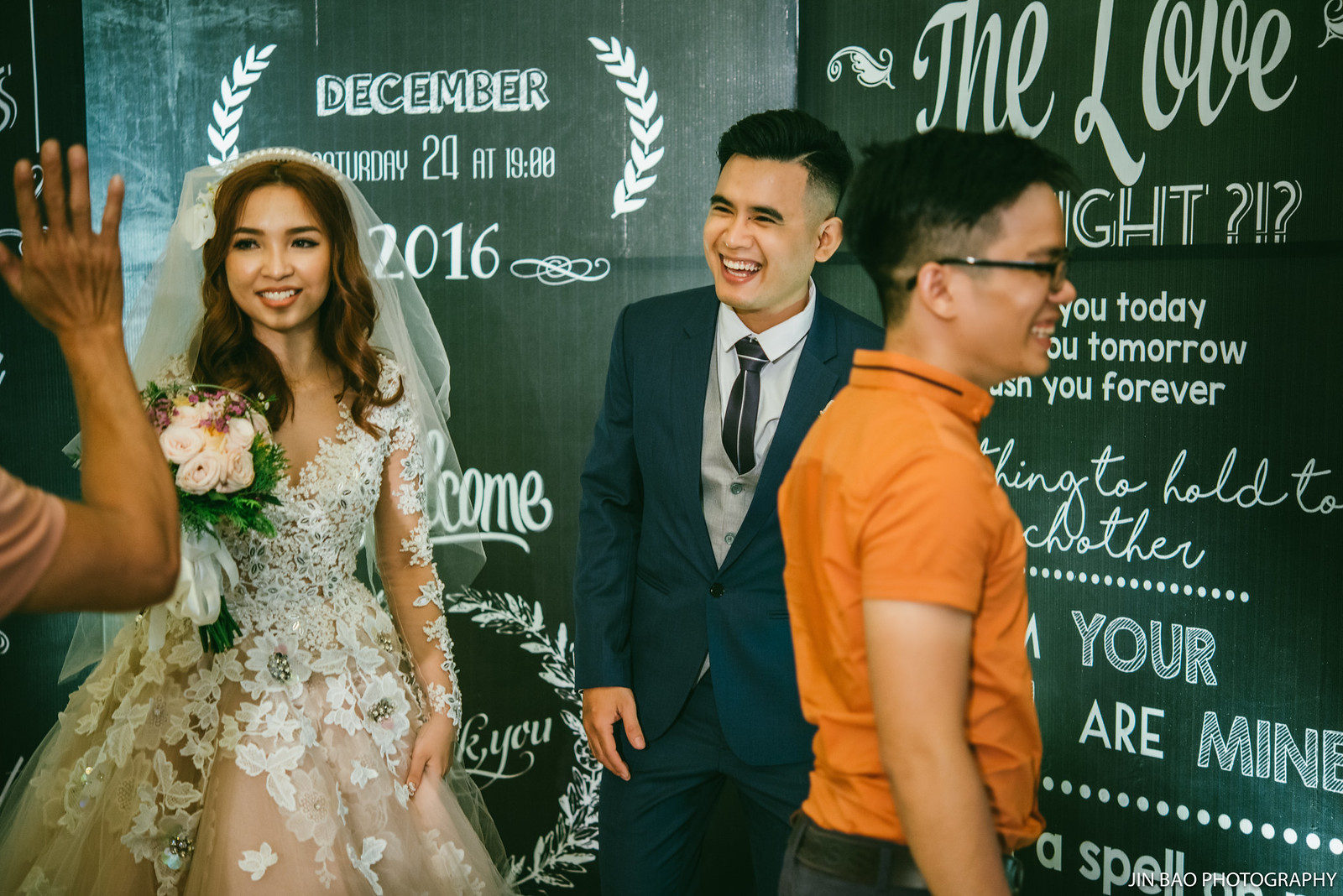This is an informal photograph capturing a joyful moment at a wedding. The focal point is the bride and groom, who are gazing happily at an off-camera person whose arm, elbow, and hand are visible in the frame, with the hand raised up and all five fingers extended. The bride, with long brown hair, is radiant in a white gown complete with a veil and a bouquet of flowers. Beside her, the groom beams in a dark suit complemented by a gray vest and dark tie. Both are smiling broadly, reflecting the joy of the occasion.

To the right of the couple stands another man, laughing heartily and looking towards the right. He is attired in an orange short-sleeved shirt, dark pants, and dark glasses, and his face exhibits a full, toothy smile. 

Behind them, two large blackboards serve as a backdrop, covered in chalk writing. Key phrases such as "December, Saturday 24 at 1900, 2016," "welcome," and "today, tomorrow, you, forever," are visible, though some words are obscured by the people in the foreground. The setting captures the lively atmosphere and the sense of togetherness on this special day.